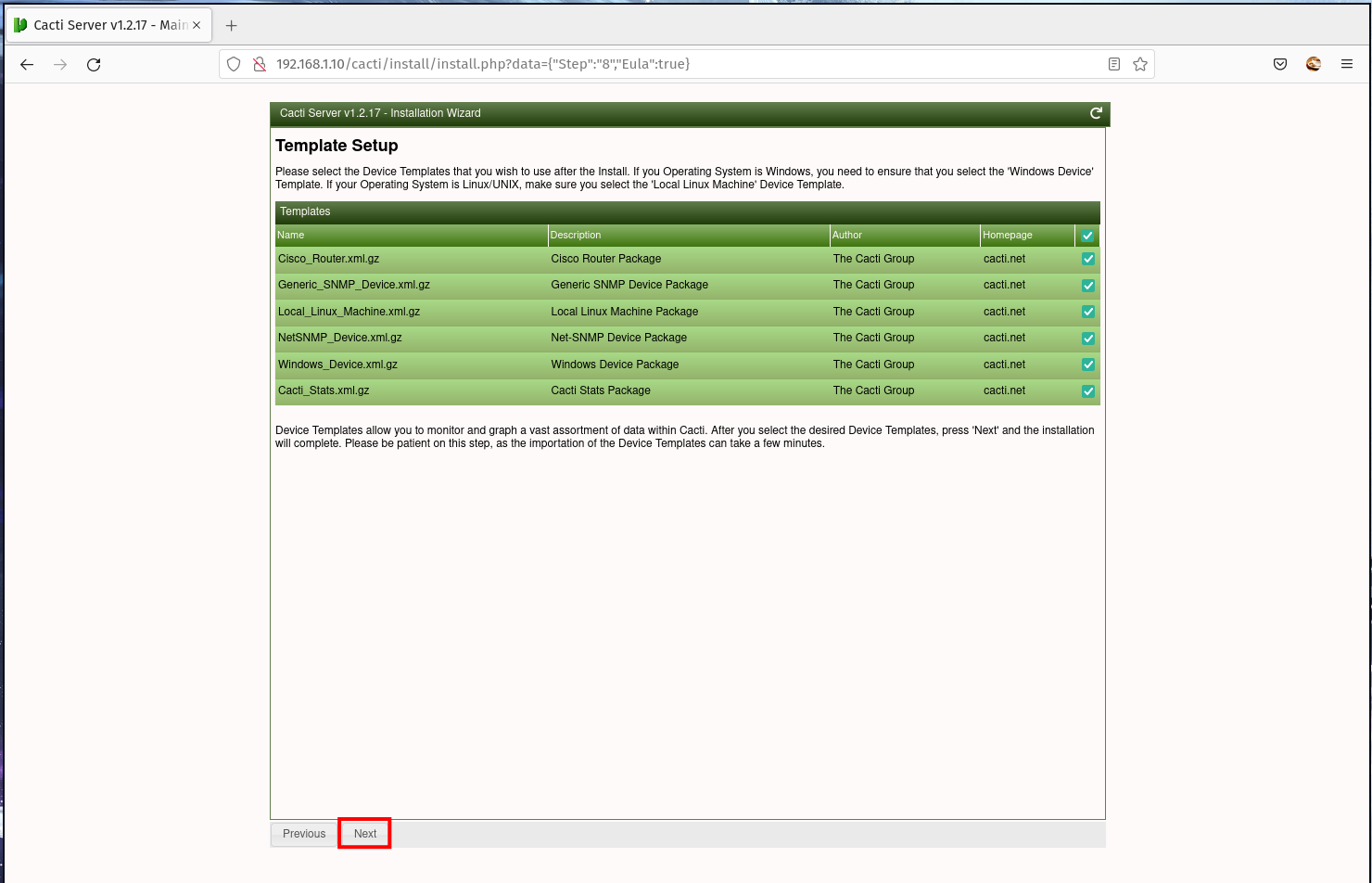A detailed caption for the given image:

The screenshot displays a web-based control panel for the Cacti Server v1.2.17 installation wizard, accessed via a private server at the URL 192.168.1.0/cacti/install/install.php?data=[]step. The interface design resembles a typical webpage with a tab at the top left corner labeled "Cacti Server v1.2.17." The main installation wizard box is centered prominently on the screen, featuring a dark green header titled "Template Setup" in black text on a white background. Below this, another dark green header labeled "Templates" introduces a section where users can select from various template options. The available options listed include "Name," "User Plan," "Author," with specific templates like "Cisco Router," "Generic SNMP," and "Local Linux," which cater to different network configurations. A detailed description informs users that device templates allow for monitoring and graphing a broad range of data within Cacti. Users are instructed to select the desired device template and press "Next" to complete the installation. It notes that the importation of device templates may take a few minutes, emphasizing the importance of patience during this step. At the bottom of the wizard box, there are navigation buttons labeled "Previous" and "Next," with the "Next" button highlighted in red for emphasis.